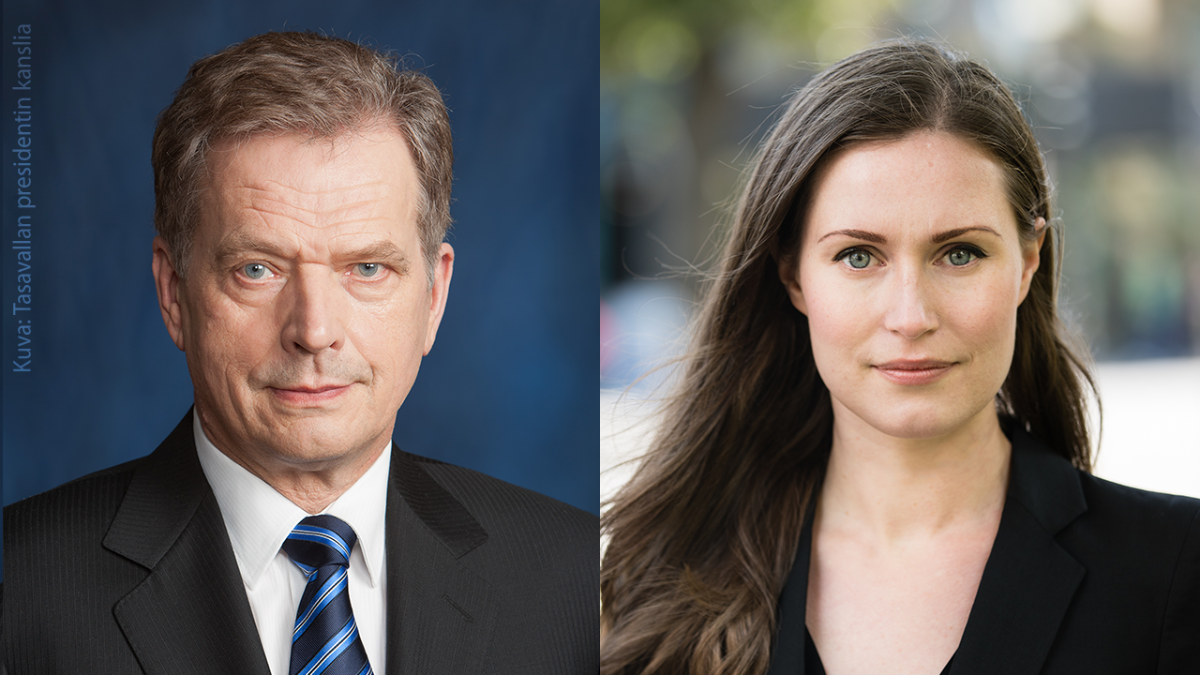The image consists of two side-by-side professional photographs, each featuring a distinct individual. On the left is a middle-aged man, likely in his 50s or 60s, with short brown hair and blue eyes. He is dressed in a black sport coat, a white shirt, and a blue tie with light blue stripes. The backdrop behind him is a solid dark blue, contributing to the formal tone of the image. Text on his side reads "Kuva Tassavallan Presidentin Kansila," suggesting some official context.

On the right is a woman with long brown hair, light blue eyes, and a pale complexion. She is dressed in a black blazer, and like the man, is visible from the chest up. Her background is significantly blurred, though there seems to be a suggestion of a cityscape or park behind her. The softer focus contrasts with the clear, solid backdrop of the left photograph, yet both images convey a sense of professionalism and formality.